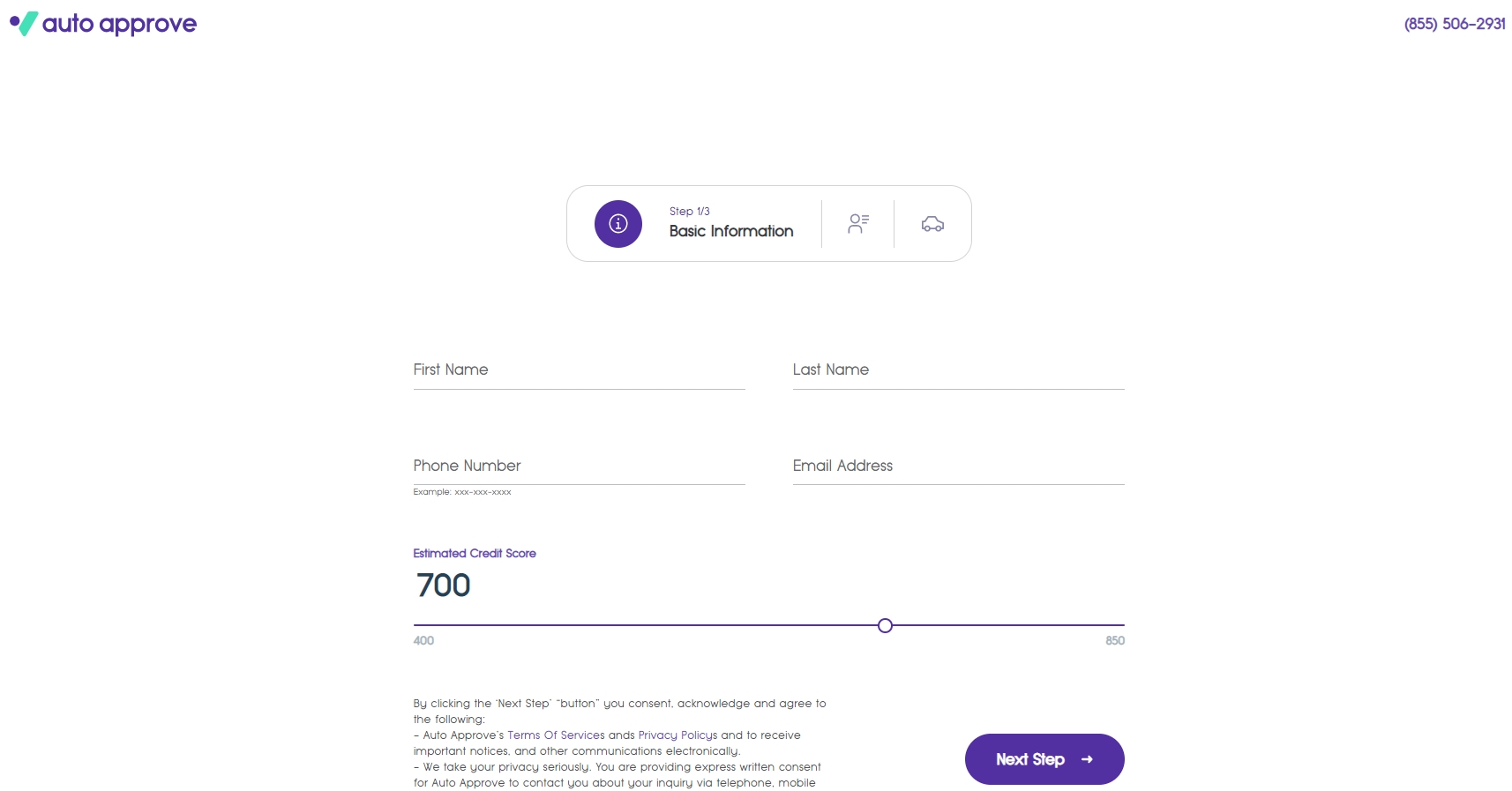The image depicts a website interface for a service called "auto-approve." At the top of the webpage, there's a distinctive logo consisting of a purple dot or circle with a green line running diagonally from the top right to the bottom left. The name "auto-approve" is displayed in lowercase letters in purple text next to the logo. On the right side of the header, there is a customer service phone number presented in purple text: (855) 506-2931.

The main section of the webpage features a white background. Central to this area is a square with rounded edges containing a design element—a purple circle with the letter "i" inside it. Below this, the text "Step 1 of 3: Basic Information" is printed in black. Accompanying this text is an icon resembling a simple drawing of a person (a circle for the head and an upper part of a square for the body) and a car icon.

Below these icons are several input fields with corresponding labels for users to enter their information:
- First Name
- Last Name
- Phone Number
- Email Address

Additionally, there is a field labeled "Estimate Your Credit Score," with the number 700 displayed.

At the bottom of the form, a disclaimer reads: "By clicking the 'Next Step' button, you acknowledge and agree to the following: the auto-approve's terms and conditions." A purple banner with the text "Next Step" and right-facing arrows is prominently featured, indicating the button to proceed.